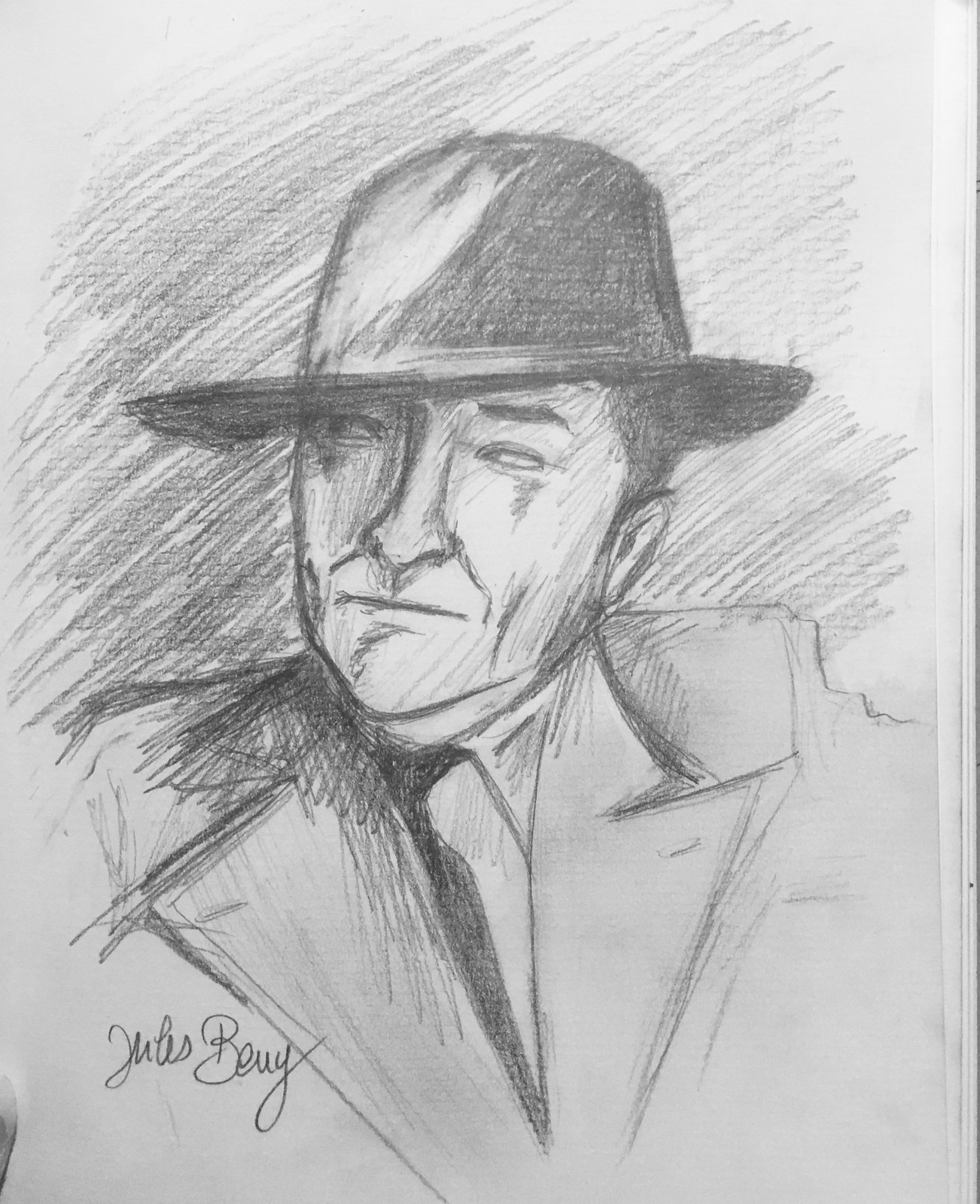The image is a detailed black and white pencil sketch of a man resembling an old-time private detective or investigator. He is wearing a dark, sharp-edged fedora hat that sits just above his eyebrows, casting a shadow on his stern and intuitive face. His facial expression is quite stern, with his left eyebrow slightly raised and his eyes looking sharply to the left, giving a sense of cautious attention. The man possesses strong, stony facial features, including a long, prominent nose and a well-defined jawline. He is dressed in a traditional business suit, complete with a black tie and possibly a suit vest underneath, hinting at his professional demeanor. The background consists of pencil-shaded lines that accentuate the detail in his form. In the bottom left-hand corner of the sketch, the artist's signature reads "Jules Bui," denoting the creator of this detailed piece of art.